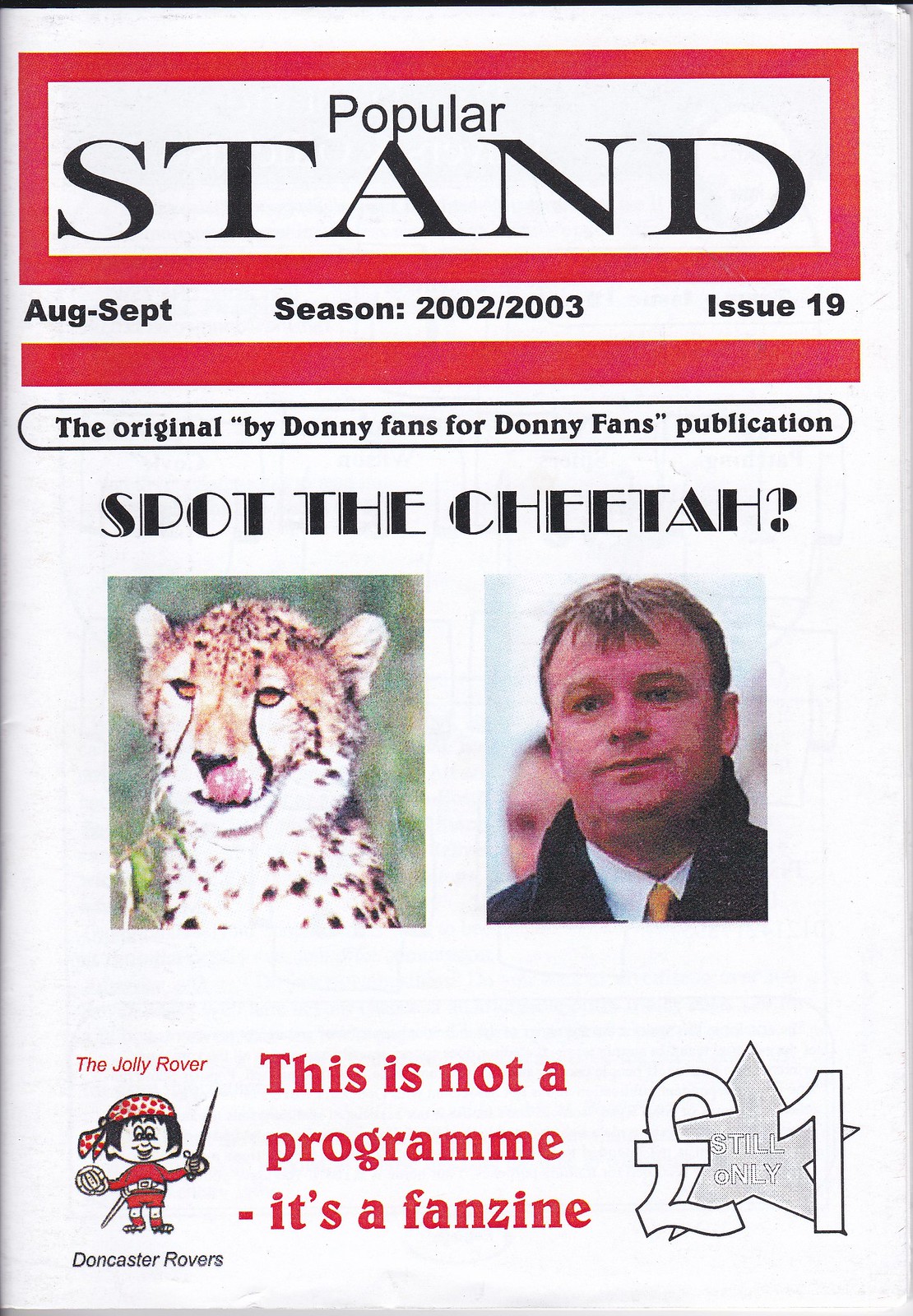This image is the cover of a fanzine, primarily featuring a white background with black letters at the top stating "Popular Stand." The header includes "August through September, Season 2002-2003" followed by "Issue 19." Just below this, inside a small box, it reads "The Original by Donnie Fans for Donnie Fans Publication." 

Centrally positioned are two prominent images: a photo of a leopard on the left and a man on the right, juxtaposed with the provocative caption "Spot the Cheetah?" in black letters. The cover color palette is mostly black, white, and red with some instances of green, orange, pink, and gray.

At the bottom, in red letters, it reads "This is not a program. It's a fanzine." Additionally, the cover mentions the cost being one euro, suggesting that this is not a typical game day program but a special, fan-created magazine for the 2002-2003 season.